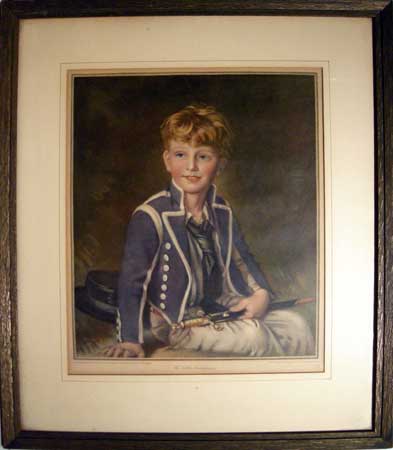This detailed portrait shows a young red-haired boy, aged around eight to ten, captured in a vintage style. The image is set in a sturdy dark brown wooden frame, with a wide ivory-colored matting that features a subtle brass liner, giving it an antique appearance. The boy, dressed in a blue, military-style jacket adorned with brass buttons and wide lapels, sits facing forward with a slight tilt of his head to the left and a cheerful smile on his face. His hair is short, with bangs, and styled longer on the top.

The background of the portrait is made up of warm brown and tan hues, with a shiny black top hat evident behind the boy, adding to the period feel of the image. He is seated, possibly on a bench, with his legs angled to the right. His right hand props him up, palm down, while his left hand rests across his lap, holding a sword horizontally. The sword features a striking gold handle, and its dark sheath has a lightly reddish tip. Completing his outfit, he wears light linen white pants. This portrait blends elements of photographic realism with the qualities of an oil painting, capturing the essence of a bygone era.